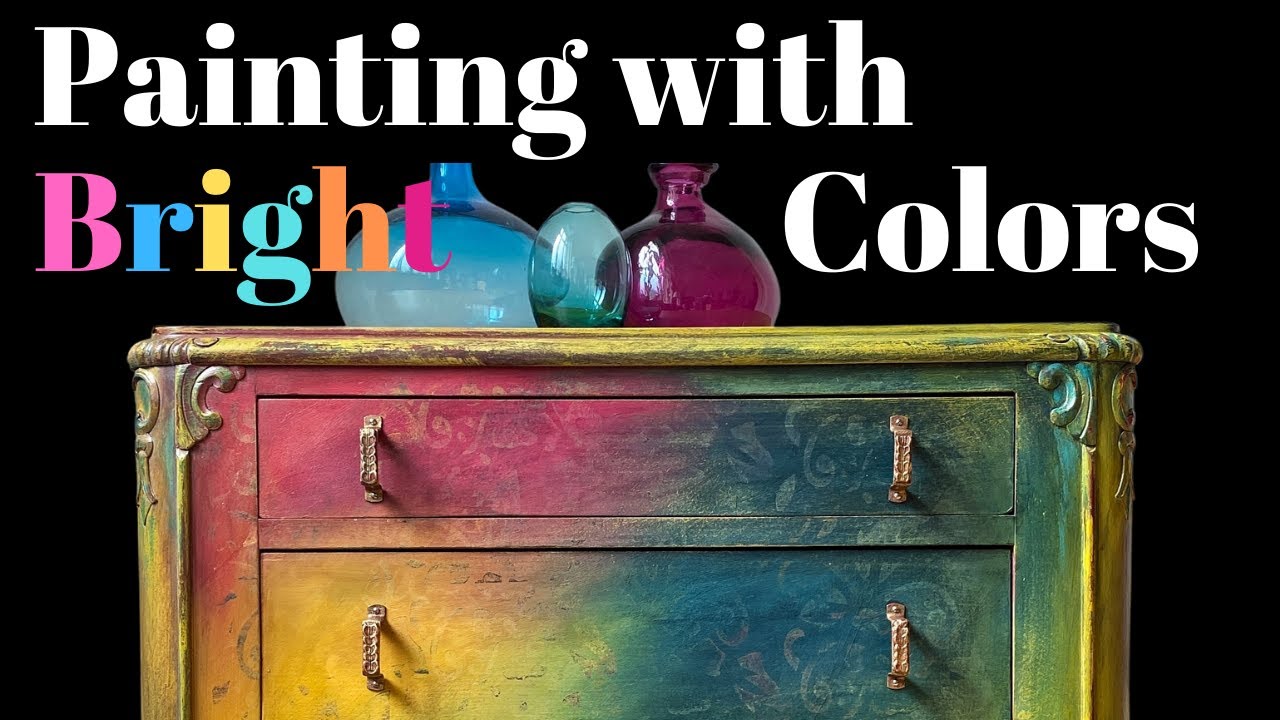This image features a horizontally-aligned, rectangular advertisement set against a stark, dark black background. Prominently displayed at the top, the text reads "painting with bright colors," where "painting with" and "colors" are written in large white letters, while "bright" is depicted with each letter in a different vibrant color. Centered in the image is a dresser beautifully painted in various sections: the top drawer is split into pink on the left and blue on the right; the middle drawer features yellow on the left and dark blue on the right; the bottom drawer combines shades of gold, red, and green. On top of the dresser sit three glass bottles of different shapes and colors: an opaque blue bottle on the left, a clear glass bottle in the middle, and a turquoise hand-blown glass bottle on the right. The overall composition effectively showcases a vivid display of bright colors against the minimalist black background, underlining the theme of the advertisement.